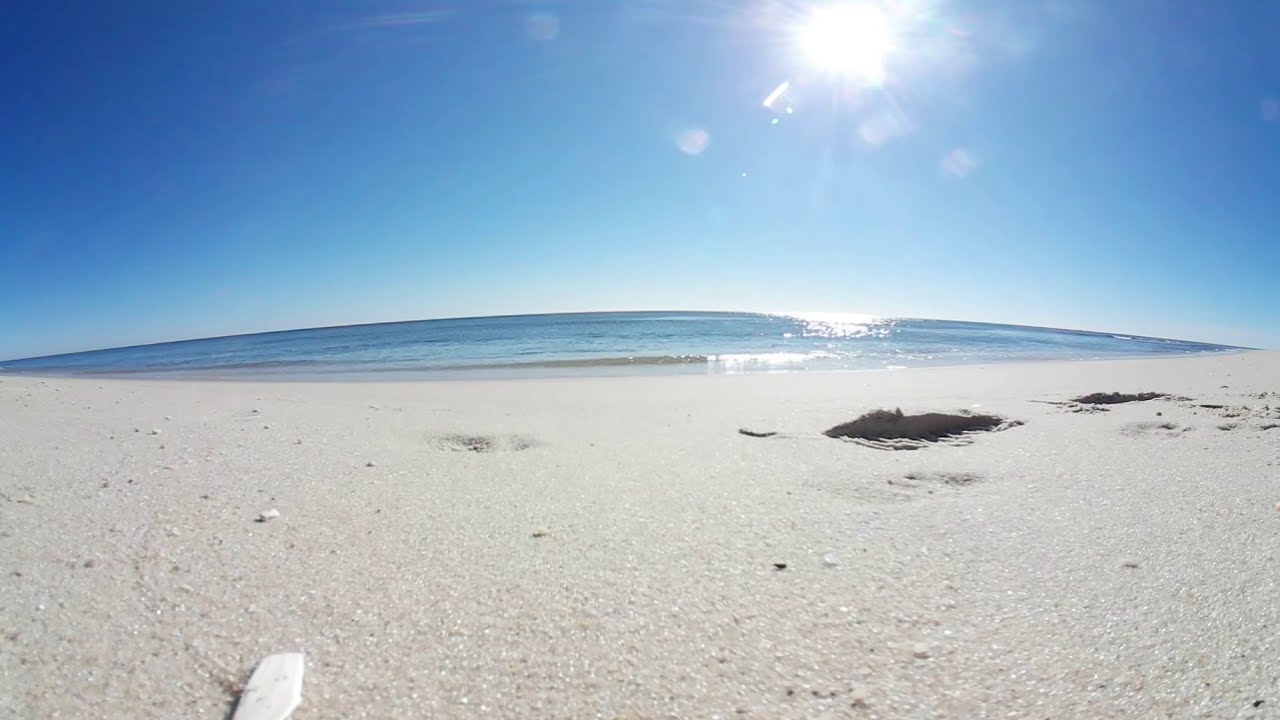A serene beach scene captured in a wide-angle photograph features a tranquil setting with flat, beige sand adorned with a few gouges and faint footprints, suggesting recent waves have swept over it. Scattered seashell fragments add texture to the serene landscape. A turquoise ocean stretches across the middle of the image, with a small wave possibly forming and sparkling under the bright sun, which is positioned toward the top right of the frame. The sun's intense light causes the water directly beneath it to glitter like white diamonds. The background showcases a clear, blue sky that gradients from light to dark. Overall, the image exudes a peaceful and calming atmosphere with its harmonious blend of sand, sea, and sky.